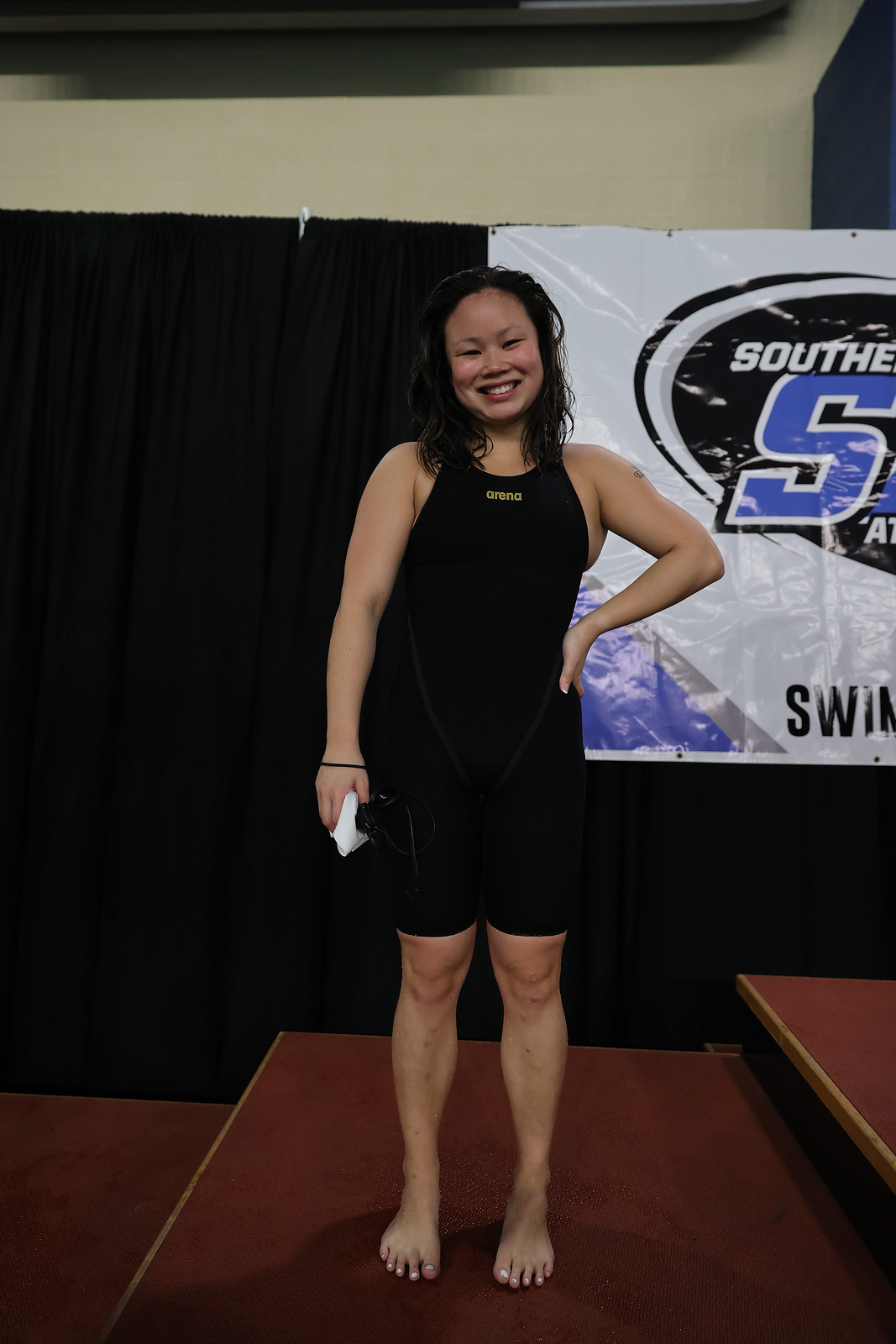In this photograph, an Asian woman stands confidently on a red, tiered platform. The platform comprises three sections that ascend from left to right, with the highest point on the viewer's right. Positioned on the middle platform, she is wearing a black racing swimsuit, sleeveless and extending almost to her knees, with the word "Arena" printed in yellow on the chest. Her outfit is complemented by her bare feet, and her hair appears somewhat wet, suggesting she has just completed a swimming event. The woman strikes a proud pose with her left hand on her hip and her right hand holding an ambiguous white item. She has long, dark hair and is smiling, radiating a sense of achievement. In the background, on the left, a black curtain can be seen, while to her right, a white banner features part of a black and blue logo and the large letter "S," possibly indicating "Southern" and hinting at an athletic event.